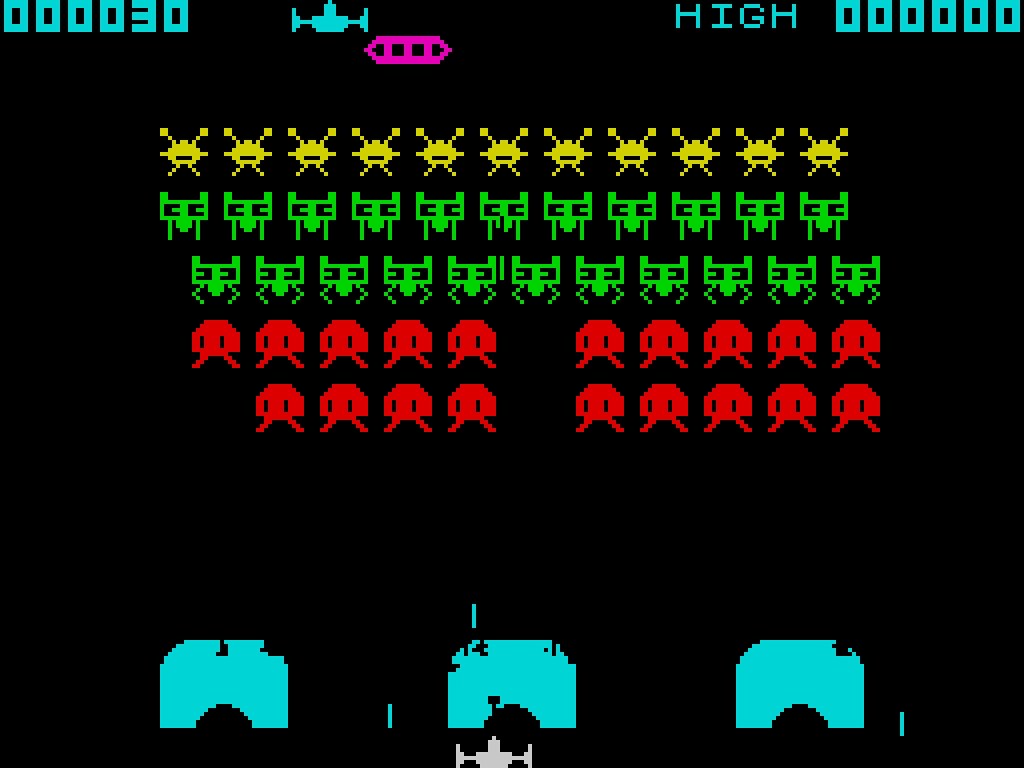This is a detailed, cleaned-up caption formulated from the provided audio description:

"A screenshot of a retro-style video game, featuring rows of alien characters. At the top of the screen, yellow X-shaped aliens are aligned, reminiscent of classic video game invaders. Below them, two distinct rows of different green-eyed aliens follow; the first row features aliens with straight legs, while the second row's aliens have bent legs at a joint. Additionally, there are red aliens with half-moon-shaped heads and V-shaped legs scattered throughout the scene. Visible in the top-left corner is the number '30,' and on the top-right, the word 'HIGH' accompanied by a series of zeros, suggesting a recent attempt or high score display in the game."